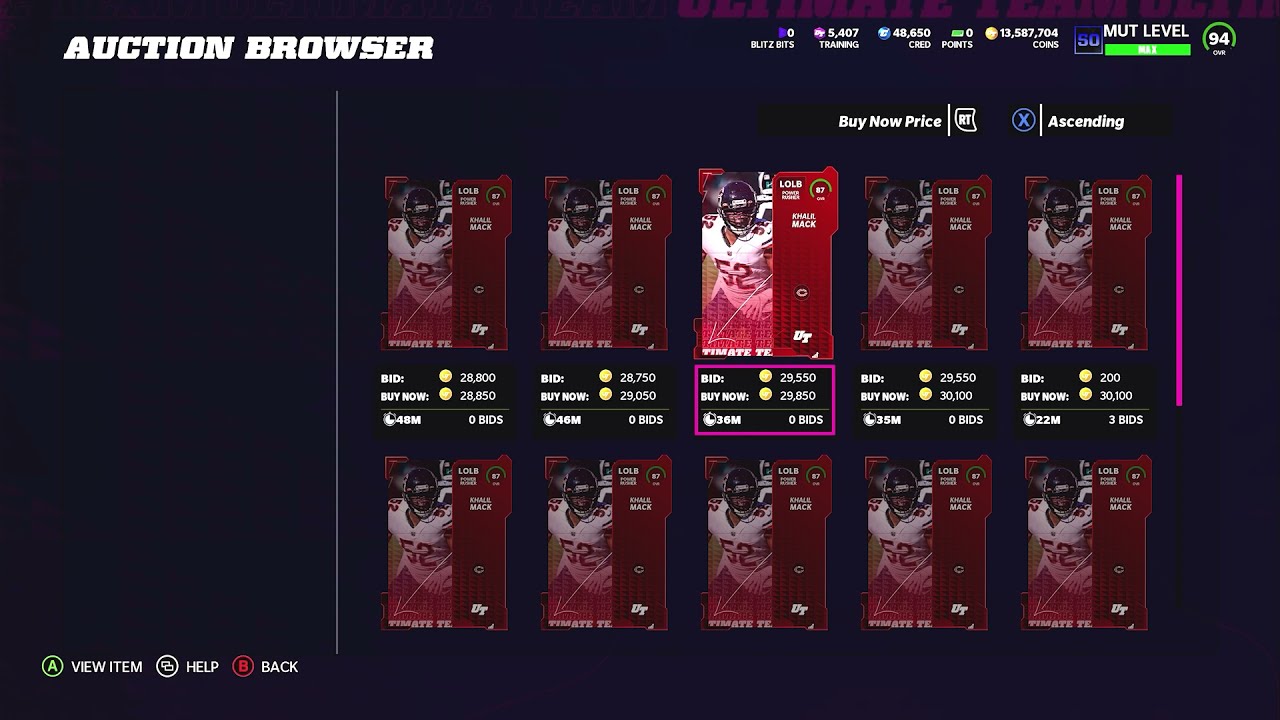This image appears to be a screenshot of an auction website, likely related to a video game, given the context and elements described. The background is predominantly black, with the phrase "Auction Browser" in white italic text located in the upper left-hand corner. In the top right corner, additional white text reads "MUT Level" followed by the number 94, and below that, "Buy Now Price," alongside the word "Ascending." A neon green bar and a circle with an X in neon blue are also visible in this section.

Beneath these headings are two rows of five panels each, showcasing a football player with jersey number 52. Each panel appears to be identical, but the center panel in the top row is highlighted with a vibrant neon pink rectangle, indicating it is the active item up for bid. This panel includes a purple box displaying options such as "Bid" with a price, "Buy Now" with another price, and possibly a timer related to the bidding process.

To the right of these panels is a conspicuous neon pink bar, while a long narrow vertical white bar is situated on the left. The lower left-hand corner of the image features white text options—"View Item," "Help," and "Back"—each accompanied by a circular icon. Specifically, "View Item" has an "A" inside its circle, "Help" contains another symbol, and "Back" includes a red icon.

Overall, the combination of these repeated elements and descriptions points to an auction system interface likely used for trading items, possibly in an online multiplayer game environment.